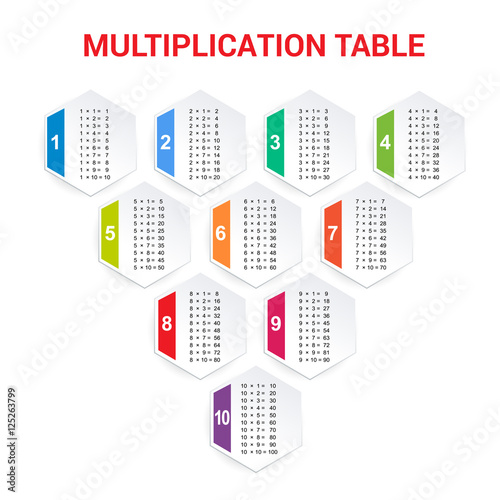The image features a meticulously organized set of multiplication tables, arranged in an upside-down triangular pattern against a white background marked with "Adobe stock" text. At the top, a prominent "MULTIPLICATION TABLE" heading appears in large, all-capital, red letters. Below the heading, there are ten hexagonal tables, each dedicated to the multiplication tables for numbers 1 through 10. These hexagons are distributed across four rows: the top row holds four hexagons, the second row contains three, the third row has two, and the bottom row has one hexagon. Each hexagon is bordered by a distinct color: blue for 1 and 2, teal for 3, green for 4, yellow-green for 5, orange for 6, red for 7 and 8, magenta-pink for 9, and purple for 10. Each colored strip is situated on the left side of the respective multiplication table, enhancing the visual distinction of each number.